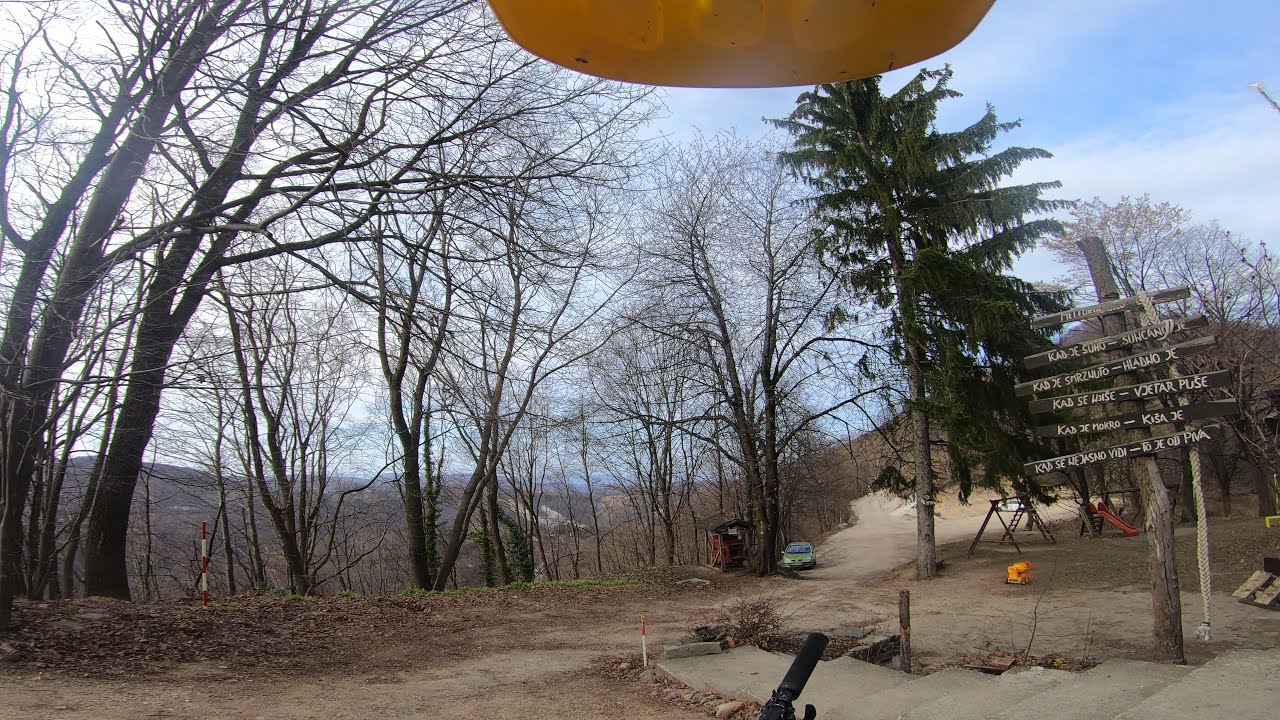The image depicts an outdoor scene on a ridge with a dirt terrain, cement steps leading down to it, and a diverse backdrop. There are multiple barren trees and evergreen pine trees, along with a small red shed and a green car parked next to a tree. In the distance, a playground features a slide, a swing set, and a yellow child's toy. A wooden signpost, constructed from a tree trunk and adorned with multiple planks, hangs nearby—its boards inscribed with destinations in a foreign language, presumably marking hiking trails. The sky above is partly sunny with blue expanses interspersed with low-flying white clouds, and the setting is amidst a mountain range, capturing a view from a high vantage point.